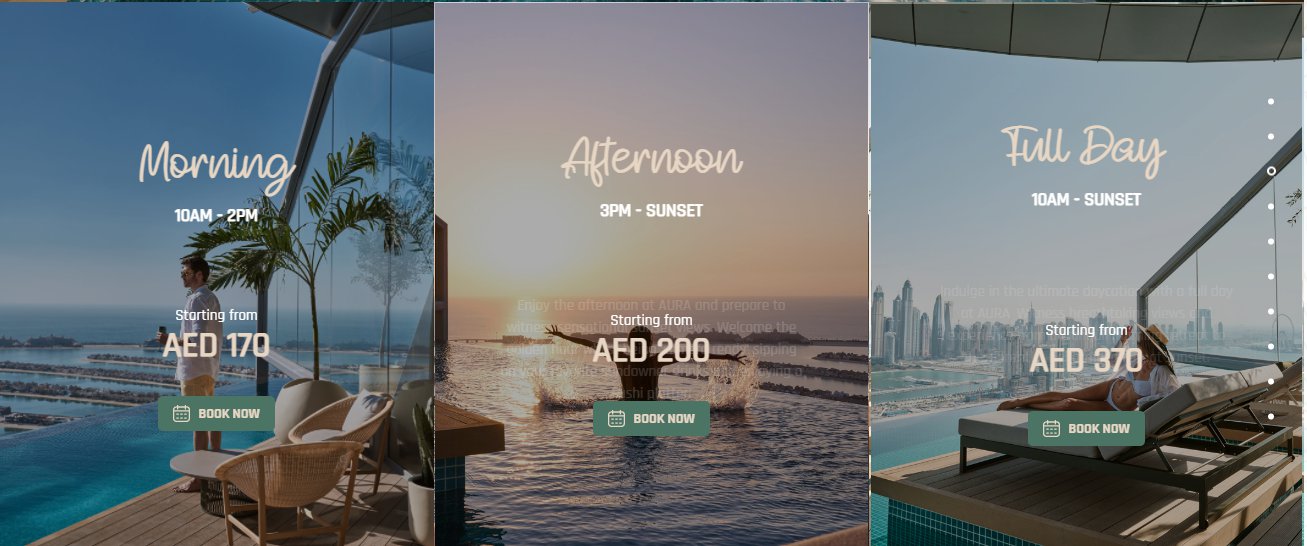The image features a triptych of promotional boxes, each detailing different vacation experiences available for booking:

1. The first box on the left depicts an individual either sitting or standing on a high level, possibly on a cruise ship, gazing out over an expansive ocean view. A palm tree and a chair are visible in the scene. The individual is wearing a shirt. Above the image, the text reads, "Morning 10 a.m. to 2 p.m. starting from AED 170." Below this image is a button labeled "Book Now," which is in a dark blue or dark green color.

2. The middle box showcases a lively scene with someone splashing in the water at the beach during the late afternoon, enhanced by the warm hues of a setting sun in the background. The accompanying text states, "Afternoon 3 p.m. to sunset starting from AED 200." Similar to the first box, there is a "Book Now" button beneath the image.

3. The rightmost box describes a full-day experience. The imagery includes a stunning city skyline under a clear sky, with a woman sunbathing in a bikini on a beach chair, wearing a hat. The text reads, "Full Day 10 a.m. to sunset starting from AED 370," and it also features a "Book Now" button below the image.

Each box offers a visual teaser of the activities available at different times of the day and their respective starting prices, encouraging immediate booking with the "Book Now" buttons.